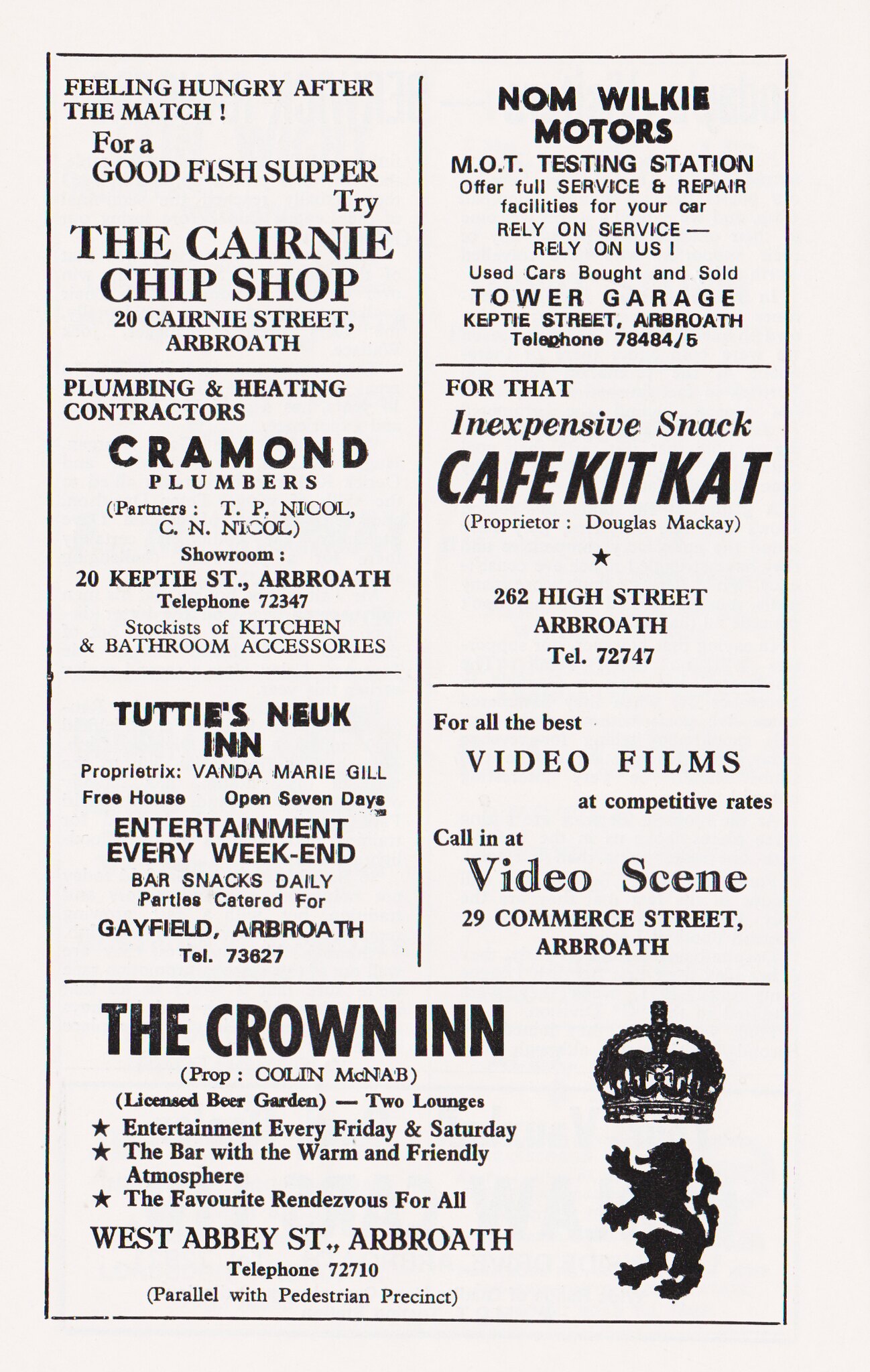This image is a scan from an insert found in a magazine or pamphlet, featuring seven black-and-white advertisements for various local businesses from Arbroath. These ads are organized within two vertical columns, surrounded by a thin black rectangular border on a white or off-white paper background. Each ad contains essential information such as the business name, address, telephone number, and service description.

At the top left, the first ad is for "The Kearney Chip Shop," located on 20 Cairney Street, promoting its fish suppers for those feeling hungry after a match. To the right of this is an ad for "Nom Wilkie Motors," a Tower Garage-based MOT testing station at Kepty Street, offering full-service and repair facilities, as well as buying and selling used cars.

Below Nom Wilkie Motors is "Cafe Kit Kat," situated at 262 High Street, advertising inexpensive snacks under the proprietorship of Douglas McKay. Left of Cafe Kit Kat is "Carmen Plumbers," plumbing and heating contractors located at 20 Kepty Street, operated by partners TP and CN Nickel, and stocking kitchen and bathroom accessories.

To the lower left is "Tuddy's Newark Inn," a Free House on Jayfield, managed by Vanda Marie Grill, which offers daily bar snacks, entertainment every weekend, and caters for parties. To the right of this is "Video Films at Competitive Rates," by Video Scene, situated at 29 Commerce Street, offering a wide selection of video films.

Dominating the bottom quadrant of the page is the largest ad for "The Crown Inn," located on West Abbey Street, and featuring a black-and-white outline of a crown with a mythical griffin-like creature beneath it. This inn, owned by Colin McNabb, boasts a licensed beer garden, two lounges, and weekly entertainment every Friday and Saturday, promoting itself as the go-to spot with a warm and friendly atmosphere.